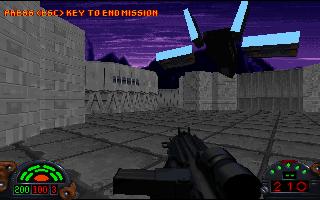The image appears to be a screenshot from a first-person shooter video game. At the top of the screen, there's a message reading "Press ESC [Esc] to End Mission," enclosed in triangular brackets around the "Esc" key. The bottom right corner of the image displays the number "210," while the bottom left corner shows "203." The perspective is from the player's point of view, with the foreground prominently featuring a gun aimed forward. The setting resembles a breezeway made of gray cement bricks for both the floor and walls, creating a maze-like environment with various pathways and places to take cover behind parts of the wall.